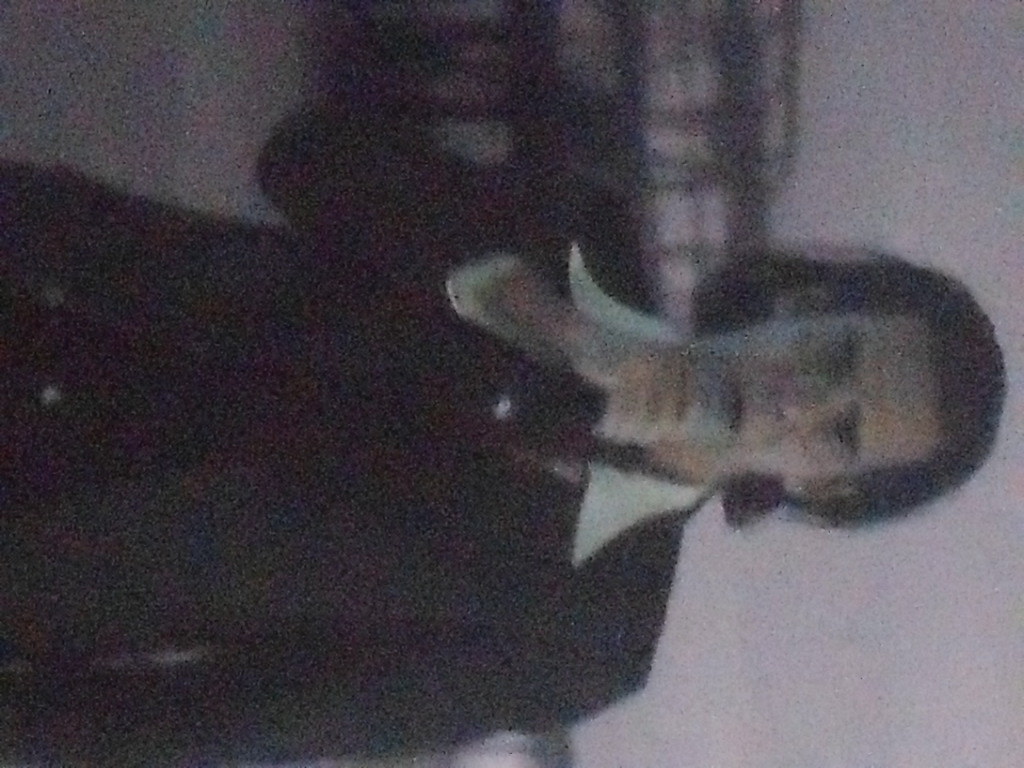The image depicts a white man standing upright, but the photograph is rotated sideways, with his head positioned to the right and his lower torso to the left. His shoulder-length, slicked-back black hair falls around his chin, and he's dressed in a black suit jacket over a wide-collared white shirt, which flares out prominently. The man appears to be holding a microphone up to his mouth with his right hand, possibly mid-song. The image is very fuzzy and out of focus, likely due to it being a low-resolution or old photograph, and the colors are extremely faint. The background is a gray color and might feature a blurry building behind him.